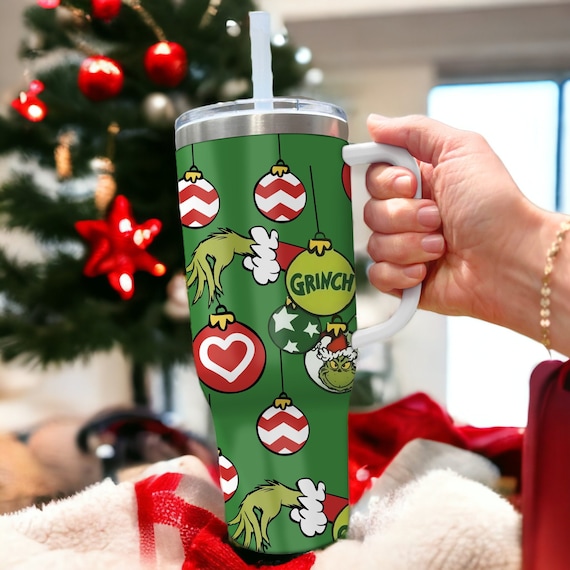This professional-grade photograph captures a festive Christmas scene featuring a prominent travel mug designed as a Thermos. The mug, adorned with an image of the Grinch holding Christmas ornaments, prominently displays the word "Grinch" in dark green with yellow accents. Its design includes a white handle, a clear lid with a metal-rimmed top, and an off-white straw.

The Thermos is held by a woman's pink-tinged hand, embellished with a gold bracelet, adding a touch of elegance to the scene. Surrounding the mug are the Grinch's green hand and red-sleeved arm with puffy white cuffs, emphasizing the Christmas theme. The mug appears to rest on a plush white blanket with hints of red plaid, contributing to the cozy holiday atmosphere.

In the background, a vibrant green Christmas tree is decorated with red stars and silver balls, set against a lush green backdrop that enhances the festive spirit. Additional ornaments, including ones with red zigzag patterns and green with white stars, hang around the scene. The composition is rich with Christmas colors—white, green, red, blue, gray, and brown—capturing the whimsical and joyous essence of the holiday season.